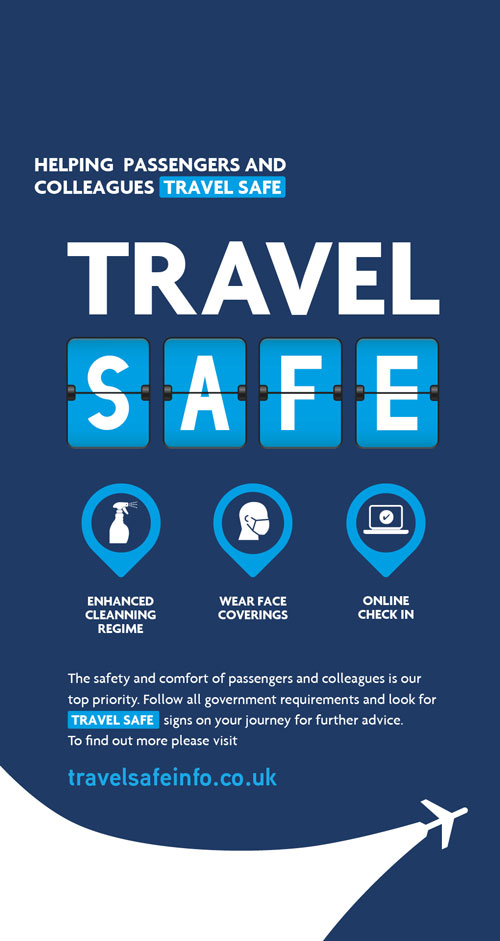The image features a rectangular design with a dark blue background. At the top, it prominently displays the text: "Helping Passengers and Colleagues Travel Safe." Directly beneath this, in larger lettering, are the words "Travel" and "Safe," styled in white text against a lighter blue background.

The center of the image showcases three adjacent icons:
1. A spray cleaner, labeled "Enhanced Cleaning Regime."
2. A person wearing a face covering, labeled "Wear Face Coverings."
3. A computer with a circle and a check mark inside it, labeled "Online Check-in."

Below the icons, an additional message states, "The safety and comfort of passengers and colleagues is our top priority. Follow all government requirements and look for Travel Safe signs on your journey for further advice. To find out more, please visit TravelSafeInfo.co.uk."

At the bottom of the image, the background transitions from dark blue to a lighter tone. Here, a white silhouette of an airplane is depicted, with a large white banner trailing behind it, giving the impression that the banner is being pulled by the aircraft.